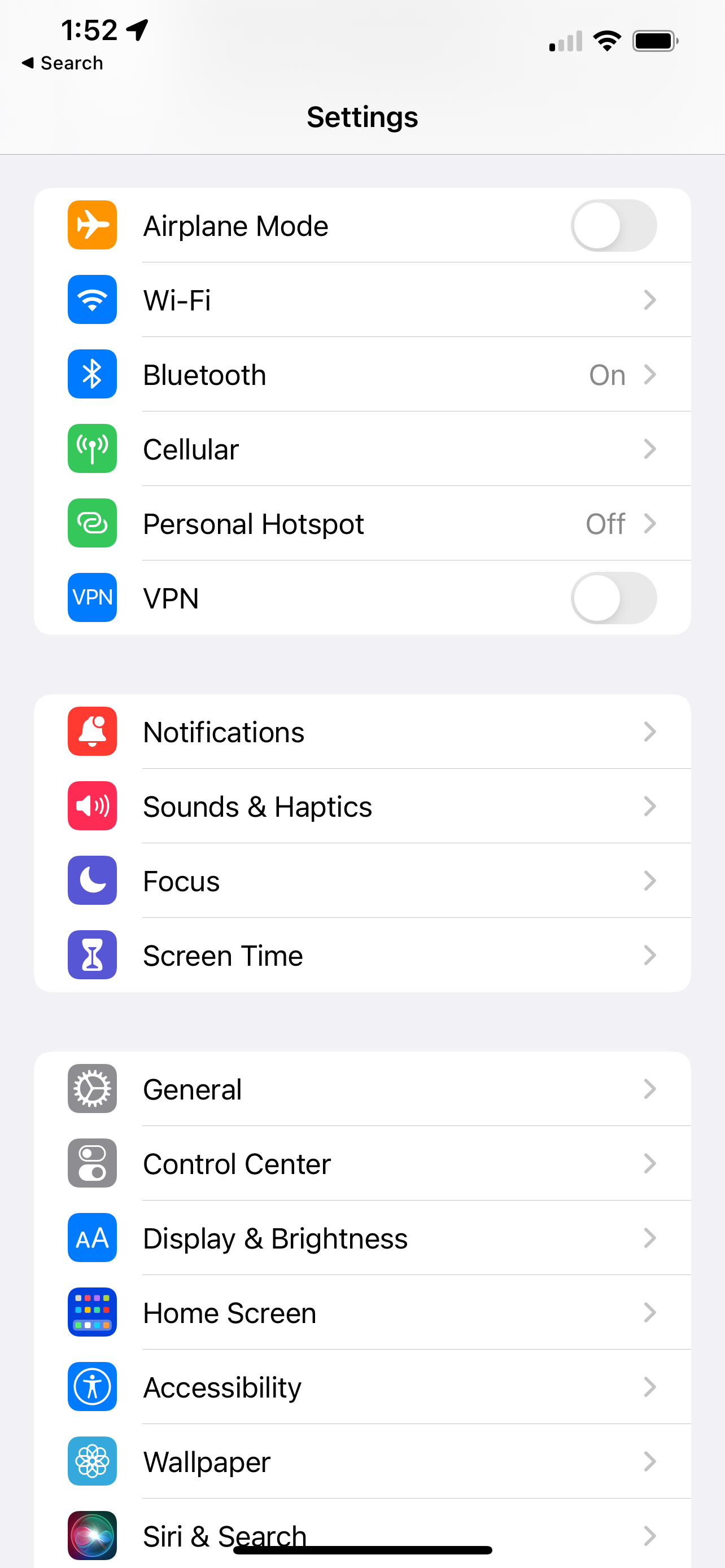The image displays the screen of a user's smartphone with a pale, grayish-blue background. At the top left corner, the time is shown as 1:52 PM, with a full battery icon and one bar of network signal to the right. Centrally positioned at the top is the word "Settings" in black text. Beneath this title, a vertical list presents various phone settings in black text, starting from "Airplane Mode," followed by "Wi-Fi," "Bluetooth," "Cellular," "Personal Hotspot," "VPN," "Notifications," "Sounds & Haptics," "Focus," "Screen Time," "General," "Control Center," "Display & Brightness," "Home Screen," "Accessibility," "Wallpaper," and "Siri & Search." The image indicates that "Airplane Mode" is turned off, "Bluetooth" is active, and "VPN" is turned off. No additional statuses for the other settings are provided in this image.